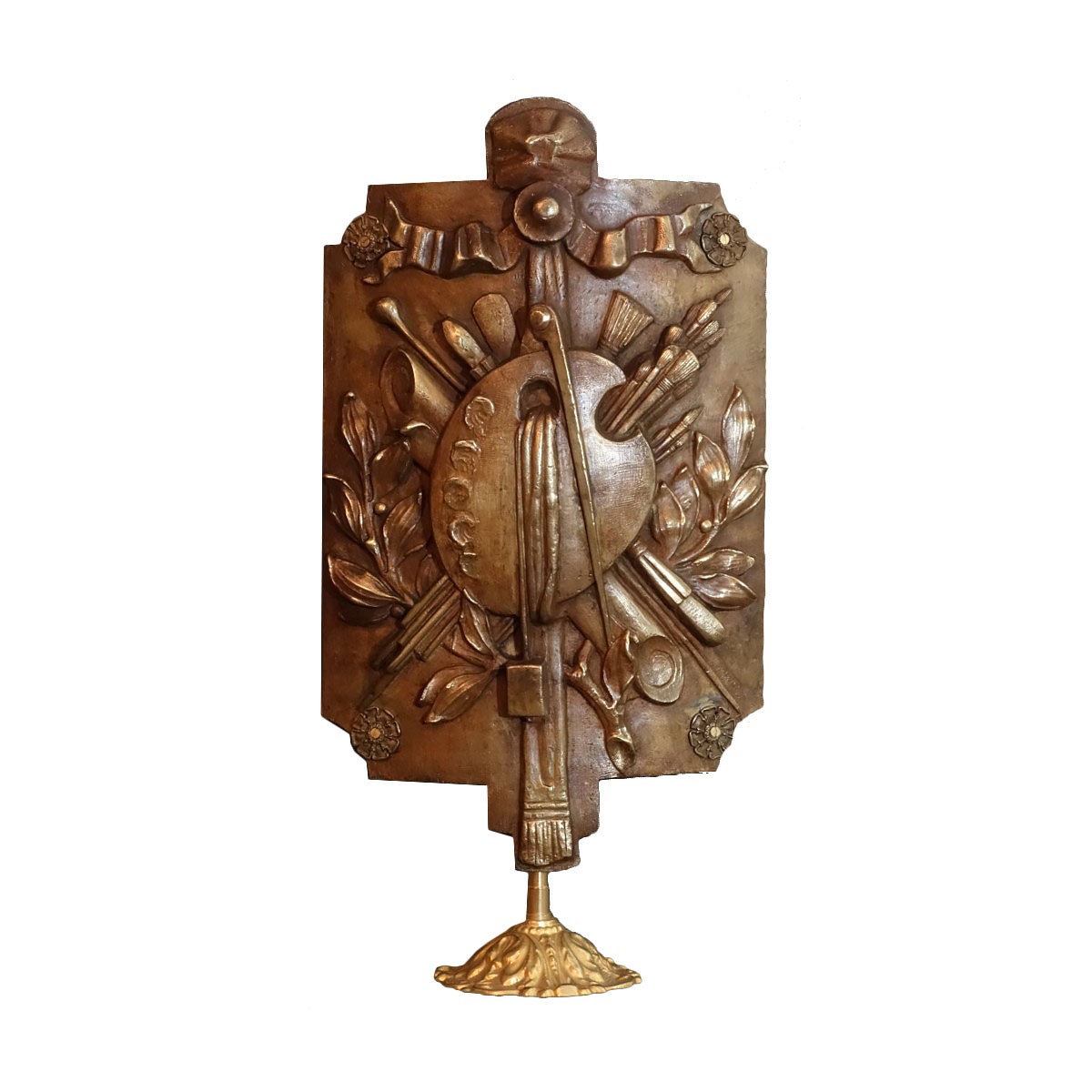Set against a white background, the image features an intricate metal artwork, predominantly coppery or bronze in color, mounted on a golden stand with a circular base and vertical pole. The artwork itself has a roughly rectangular shape with indented corners and extends vertically. Protrusions from the top and bottom edges include a stem at the bottom that transitions into a rounded, domed base. 

At the heart of the piece is an artist's palette with paintbrushes sticking out, accompanied by a drawing compass, with leafy accents behind the brushes. The upper section displays a ribbon motif that cascades into flower-like seals. Additionally, a circle with a scarf-like design extending to both sides and a smaller circle with a hole at its center enhance the overall design. The piece exudes a three-dimensional quality with a complex interplay of artistic and botanical elements.